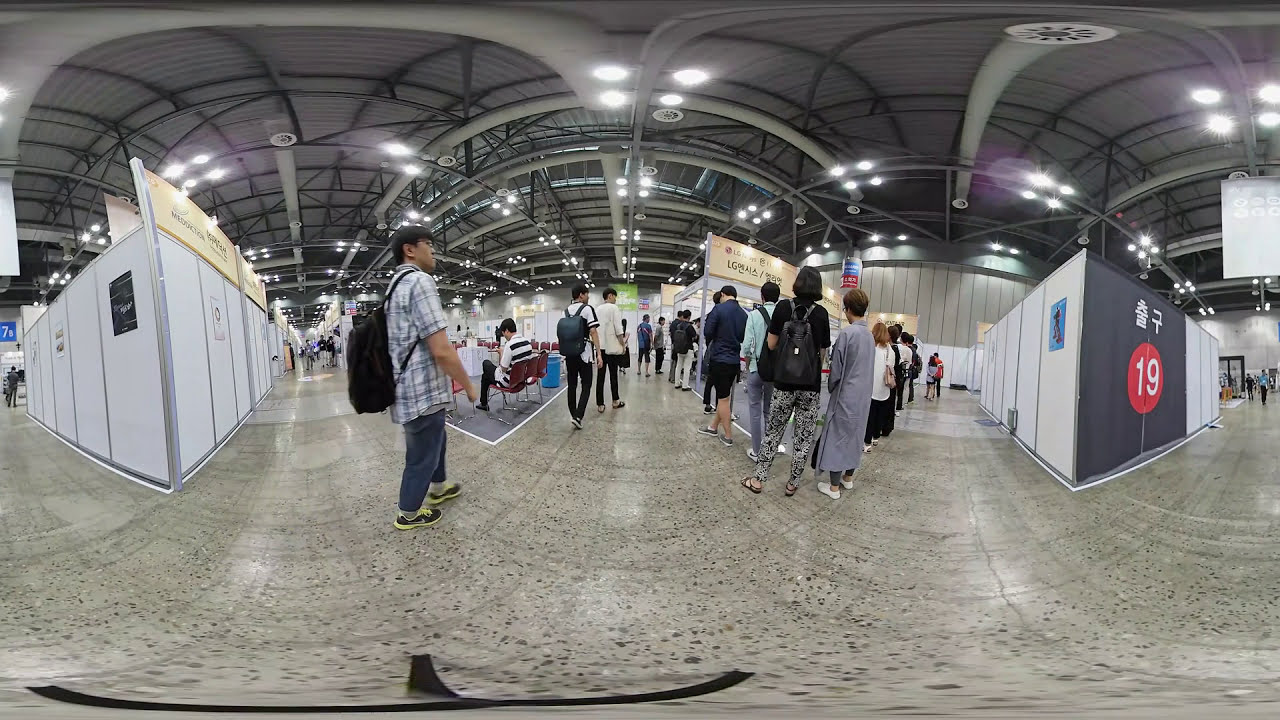The image depicts the interior of a large, curved, fisheye-lens-enhanced convention hall. The hall features a shiny gray floor with black dots, filled with people primarily seen from behind, either standing or walking, most commonly gathered towards the center right of the image. Many are carrying backpacks, suggesting they might be college or high school students. The ceiling is an intricate mesh of gray pipes and vents, adorned with numerous circular fluorescent lights that illuminate the space. The hall has several white cubicle walls on either side, likely housing various business presentations or exhibits. Some chairs are scattered around, with a few people seated. Within the cubicles, there are signs with text, possibly in Korean, adding to the informational nature of the setup.